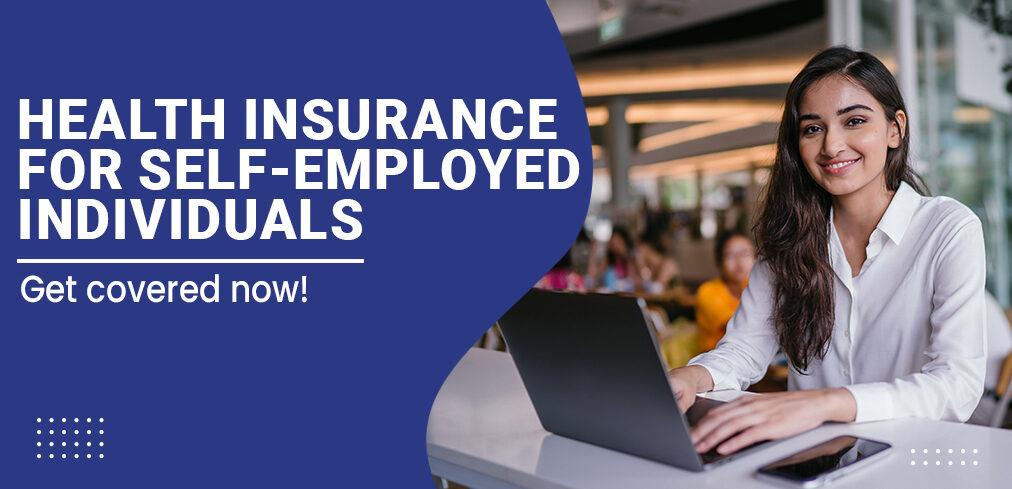This web advertisement promotes health insurance for self-employed individuals. On the left-hand side of the image, set against a blue background with white lettering, the text reads, "Health Insurance for Self-Employed Individuals - Get Covered Now." The left and right sections of the image are divided by a wavy curve. 

On the right-hand side, a woman is seated at a modern cafe, working on her laptop. She is wearing a white shirt and has long brown hair, and she is smiling as she types on the keyboard. A smartphone is placed beside her laptop on the white counter where she is sitting. The background reveals a bustling cafe environment with large glass windows that let in ample natural light, adding to the lively and contemporary atmosphere.